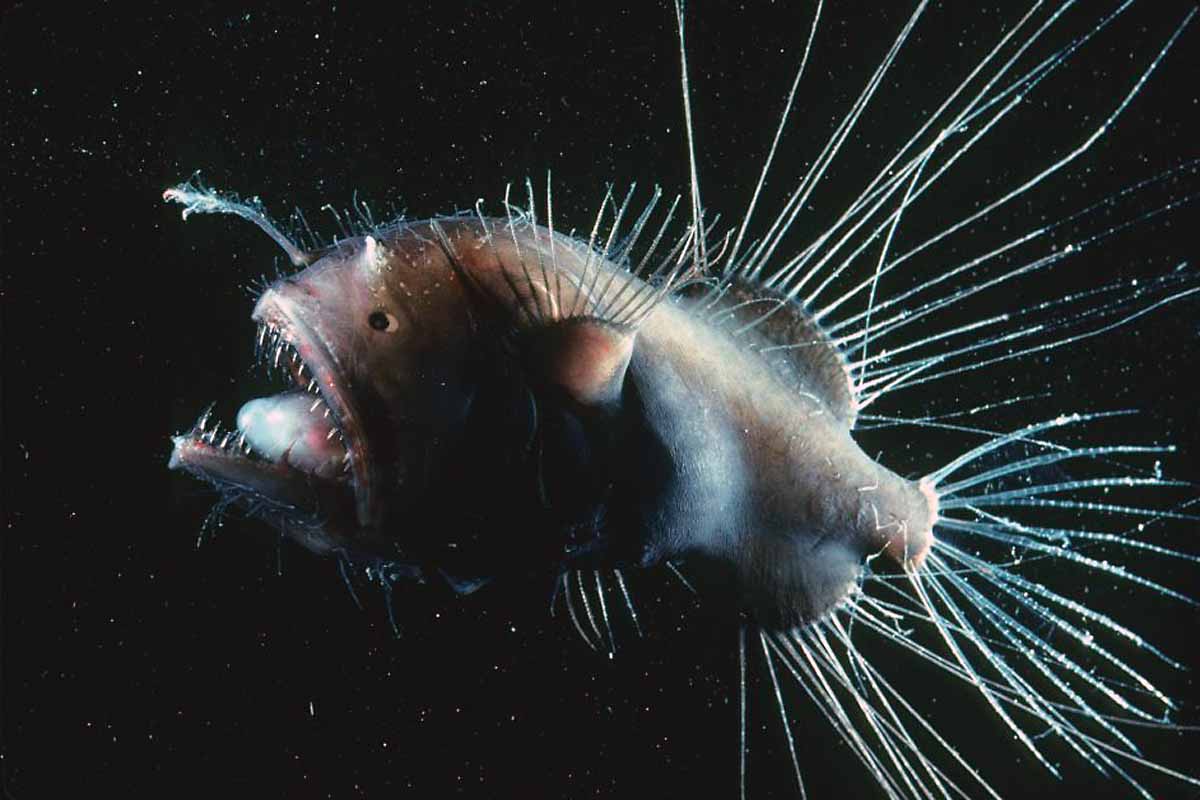In this photograph set against a black, star-speckled background, a menacing deep-sea fish takes center stage. The fish, colored in a grayish-peach hue, is dotted with numerous whitish spikes protruding from its body, giving it a fierce, almost prehistoric appearance. Its rounded form is accentuated by hair-like filaments extending from its dorsal and back areas. The creature's mouth is agape, revealing an array of sharp, pronounced teeth. Strikingly, a bioluminescent antenna-like appendage extends from its forehead, likely used to lure prey in the abyssal depths. This eerie glow is mirrored by additional bioluminescence emanating from its tail, subtly illuminating its form. The backdrop teems with tiny particles, possibly plankton, adding to the otherworldly ambiance of the scene.